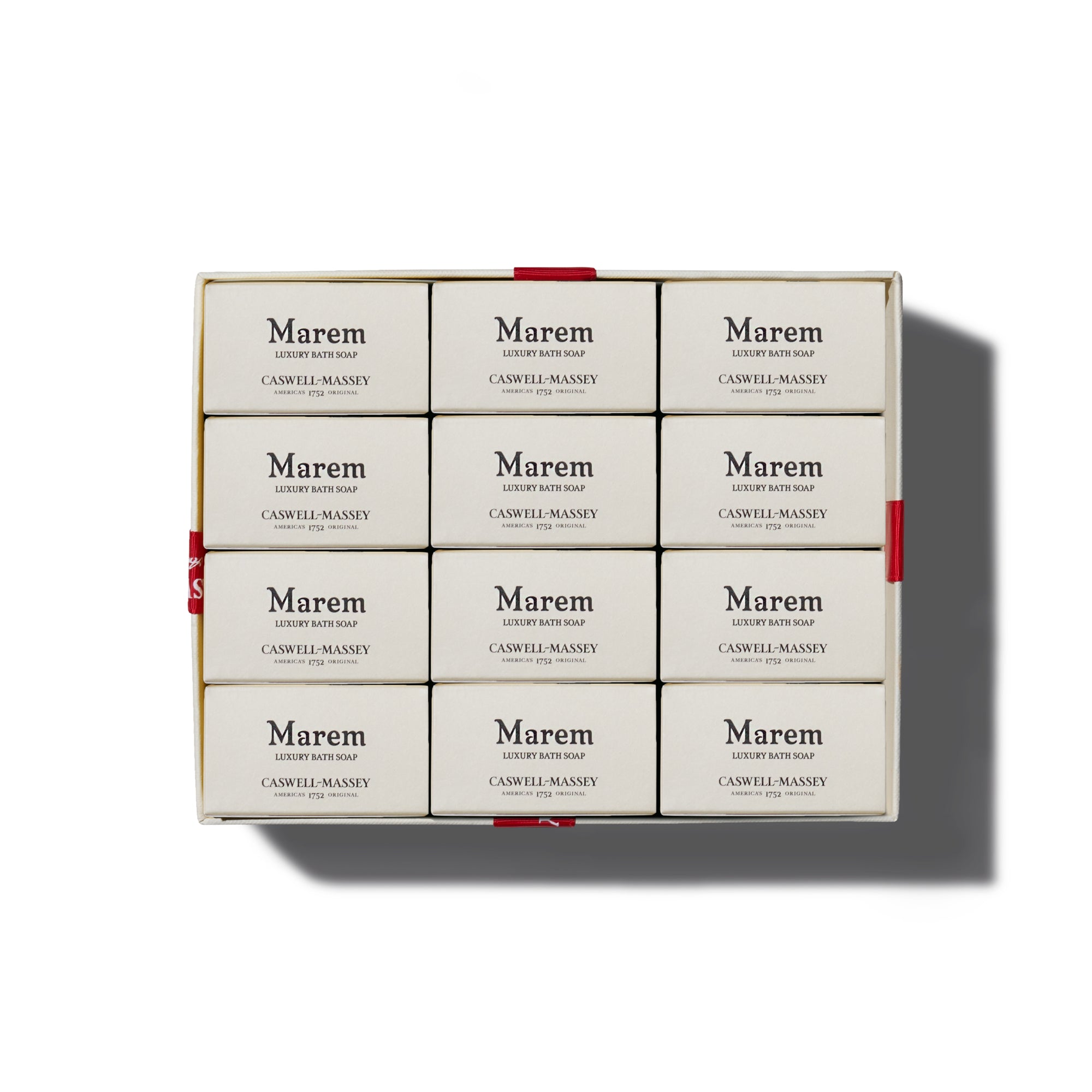This image displays an open, tan cardboard box containing 12 uniform bars of luxury bath soap, arranged in four rows of three. The box, which appears to be designed for display purposes, features red ribbons on each side that would be used if the box had a lid. Each soap bar is packaged in beige wrapping and showcases distinct black text in the center that reads "MAREM," followed by "Luxury Bath Soap" in smaller print, and "CASWELL-MASSEY" in slightly larger type beneath. The soaps are meticulously organized within the box, and the product name is centered on each bar. The entire setup, including a prominent drop shadow beneath the open box, is set against a plain white background, suggesting it is a product image likely intended for an online retail platform.